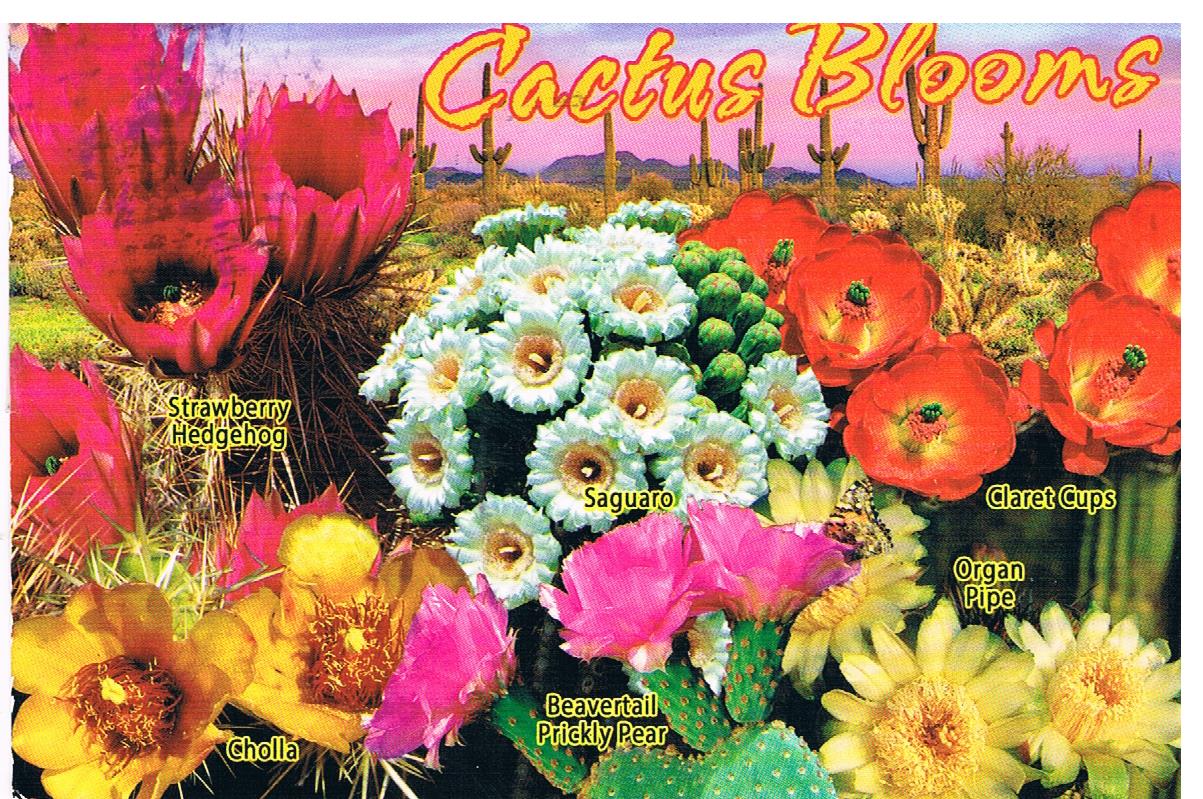In the photograph, which appears to be an advertisement for flowers, the background features a distant sky with pinks, blues, grey, yellow, and white clouds, framed by hills and cactuses. Dominating the top of the image, a prominent yellow text with a red-orange outline reads "Cactus Blooms."

Beneath this text are a series of labeled flower bouquets arranged in a grid. At the top left corner, vibrant red flowers are identified as "Strawberry Hedgehog." Directly below them, a bouquet of yellow flowers is labeled "Chola." In the center, white daisy-like flowers are marked as "Saguaro," and beneath them, a prickly green cactus with pink blooms is named "Beavertail Prickly Pear." To the right, at the top, orange flowers are titled "Claret Cups," and directly beneath them, another bouquet of yellow flowers is labeled "Organ Pipe."

This image effectively combines the visual appeal of various cactus flowers with clear, informative labels, set against a picturesque, natural backdrop.